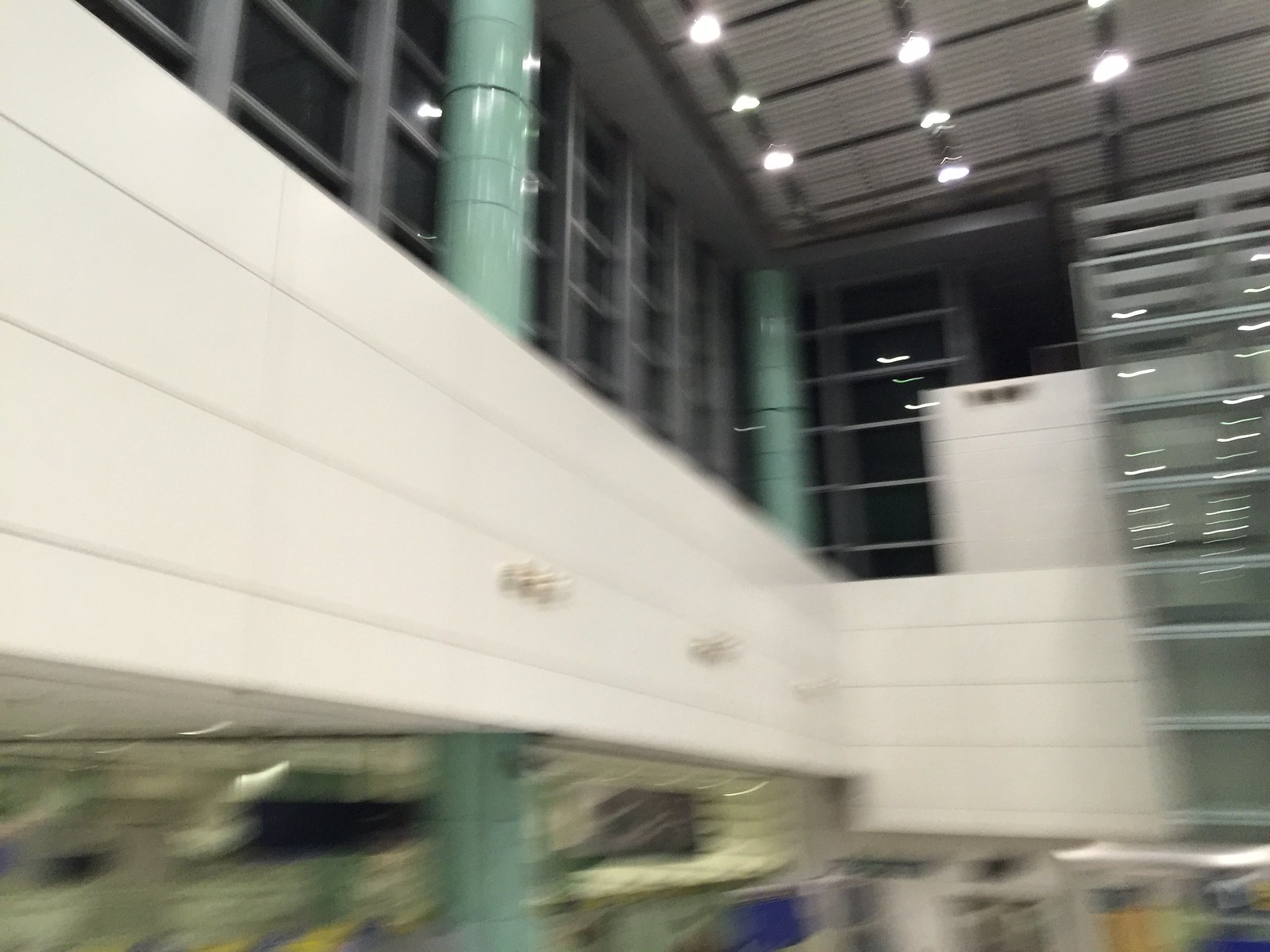A very blurry photograph taken inside a building, possibly a factory, capturing the view upwards towards an upper level. The ceiling, composed of gray square panels with black lines dividing them, features white lights at each corner of the squares. On the left side of the image, an upper-level wall with windows is partially visible, with another window around a corner obscured by stacks of unidentified items. The scene is intersected by two light blue cylindrical poles, positioned approximately one-third from the left and slightly beyond the middle of the image. A large, white, rectangular tunnel-like structure runs along the wall, turning a corner and extending further until it meets the stacked objects. The lower part of the image remains too blurry to discern additional details.